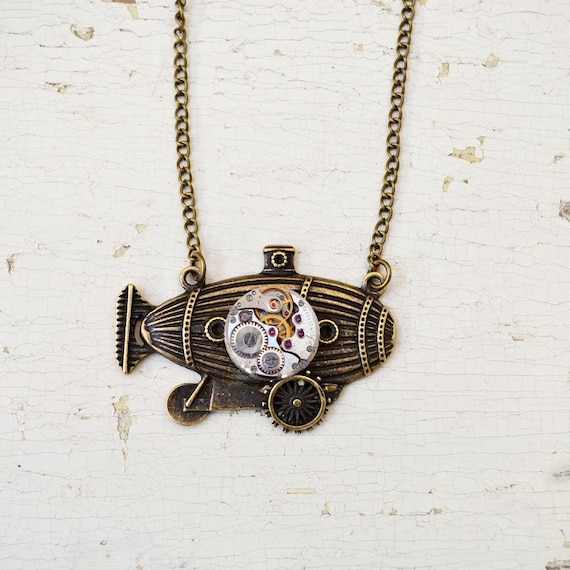This image depicts a vintage necklace featuring a large pendant shaped like a dirigible or airship, likely resembling a blimp. The pendant, which appears worn and tarnished, suggesting age or frequent use, is suspended from a dull, dark-colored metal chain. The airship-shaped pendant is black with gold stripes and features a white circular dial at its center, adorned with small cog wheels and an orange object, possibly indicating a steampunk aesthetic. Notably, the pendant includes two wheels at the bottom and a dorsal fin at the back, enhancing its airship resemblance. The pendant has a small upward protrusion at the top, completing its detailed and intricate design.